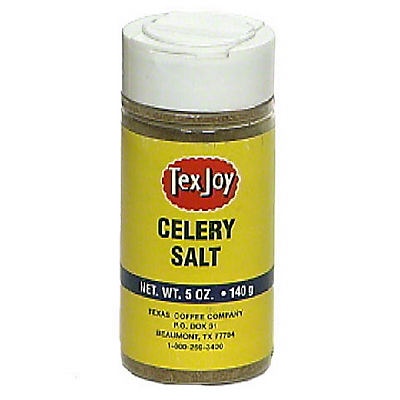This image shows a container of celery salt centered against a solid white background. The container is cylindrical with a white flip-top cap. The clear container reveals the brown celery salt inside. The label, which covers most of the container, is bright yellow. At the top of the label, the brand name "TexJoy" is prominently displayed in white letters, encircled by a squiggly line outlined in white. Below that, in large black capital letters over two lines, it says "CELERY SALT." Further down, a small black strip details the net weight as "5 ounces (140 grams)." At the bottom of the label, in small black print, it reads: "Texas Coffee Company, P.O. Box 51, Beaumont, Texas, 77704," along with the phone number. The design and labeling make it clear that this is a jar of TexJoy celery salt.